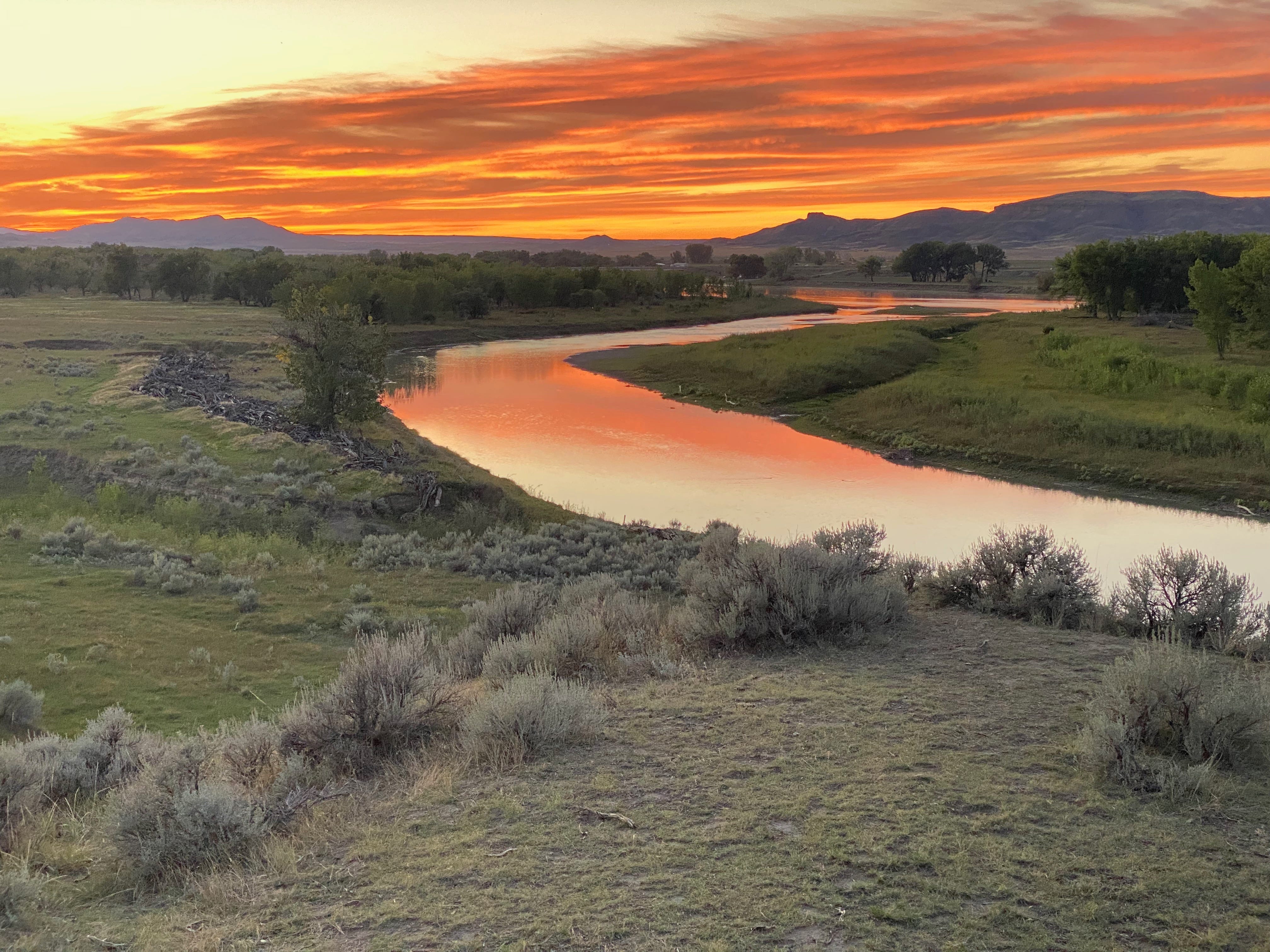This captivating outdoor photograph showcases a tranquil landscape during sunset. In the foreground, the ground is sparse with very short, almost ravaged grass, interspersed with dry and desiccated bushy tufts of light green and gray. The bottom of the photograph reveals patches of slightly darker green grass to the left, while scattered bushes and plants in varying shades of green extend across the scene. Dominating the middle of the image is a serene river, curving gracefully from the right middle toward the back, reflecting the vivid orange and gold hues of the sky, which suggest a mesmerizing sunset with swirling colors reminiscent of molten lava. This river appears wide initially, creating a Z-shaped curve as it narrows and bends around greener areas. Alongside the river, stretches of greenery and small bushes add texture and depth, with clusters of dark green trees framing the middle and right sections of the photograph. In the distance, a line of mountains silhouette against the fiery sky, appearing as dark purples and blacks, their peaks high on the edges and dipping toward the middle. The ethereal sky, filled with brilliant orange, yellow, and white hues, flawlessly mirrors in the calm river below, creating a harmonious and visually fascinating composition that beautifully pulls the viewer into this serene and natural landscape.